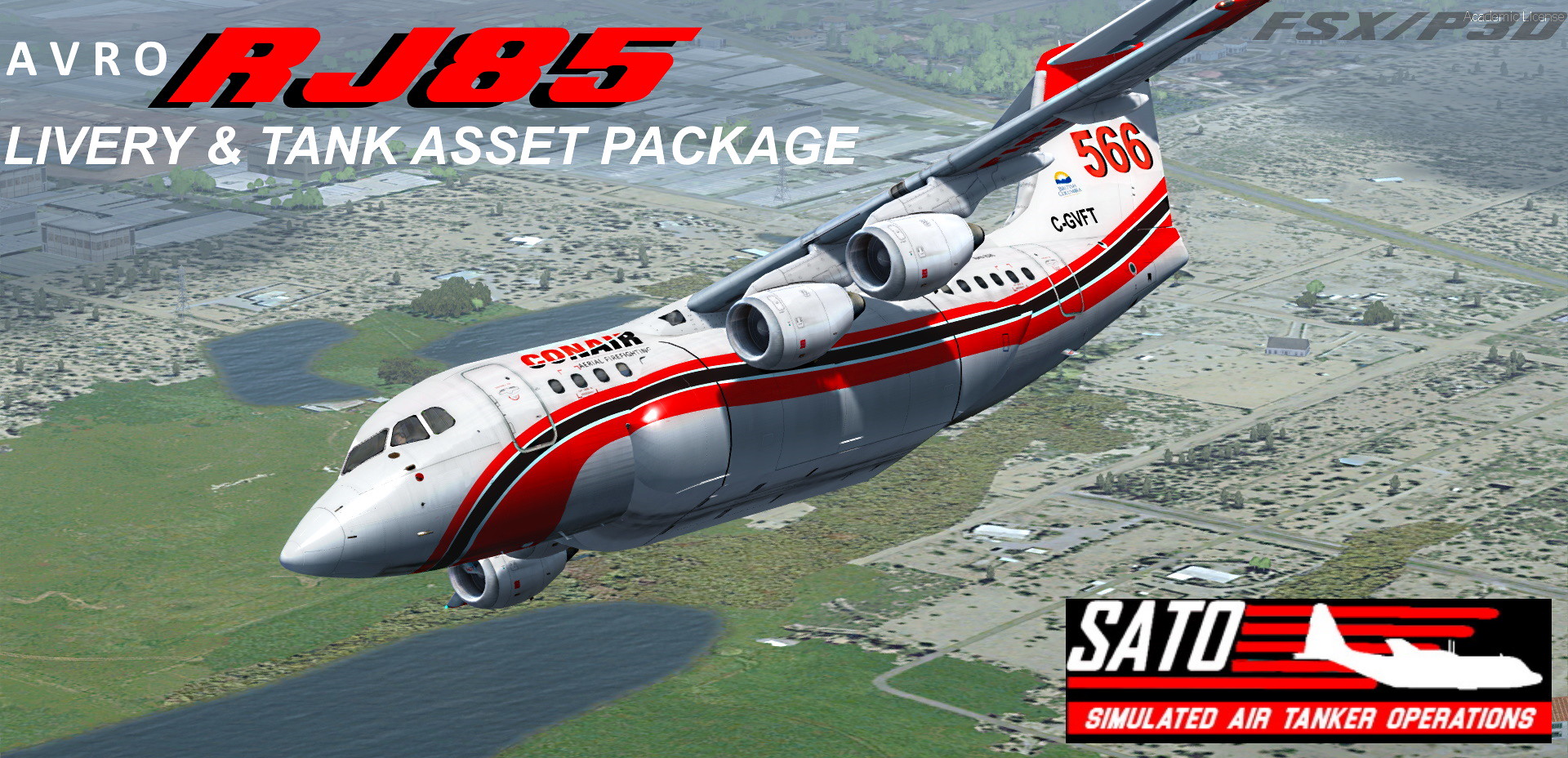The image is a detailed, computer-generated screenshot featuring a large passenger jet flying above a cityscape. The airplane, predominantly light gray in color, has a distinctive, swirly red stripe running along its fuselage. The tail of the plane is marked with the number "566" in red, while near the cockpit, the word "Conair" is clearly visible. Text in the top left corner of the image reads "AVRO RJ85" in red, followed by "LIVERY and TANK ASSET PACKAGE" in white. In the bottom right corner, there is a logo that includes the acronym "SATO" (Simulated Air Tanker Operations) with a symbol of an airplane. The airplane is centrally positioned in the image, emphasizing its importance. The green landscape below and the clear depiction of the city provide an aerial view, enhancing the realism of the simulated advertisement.